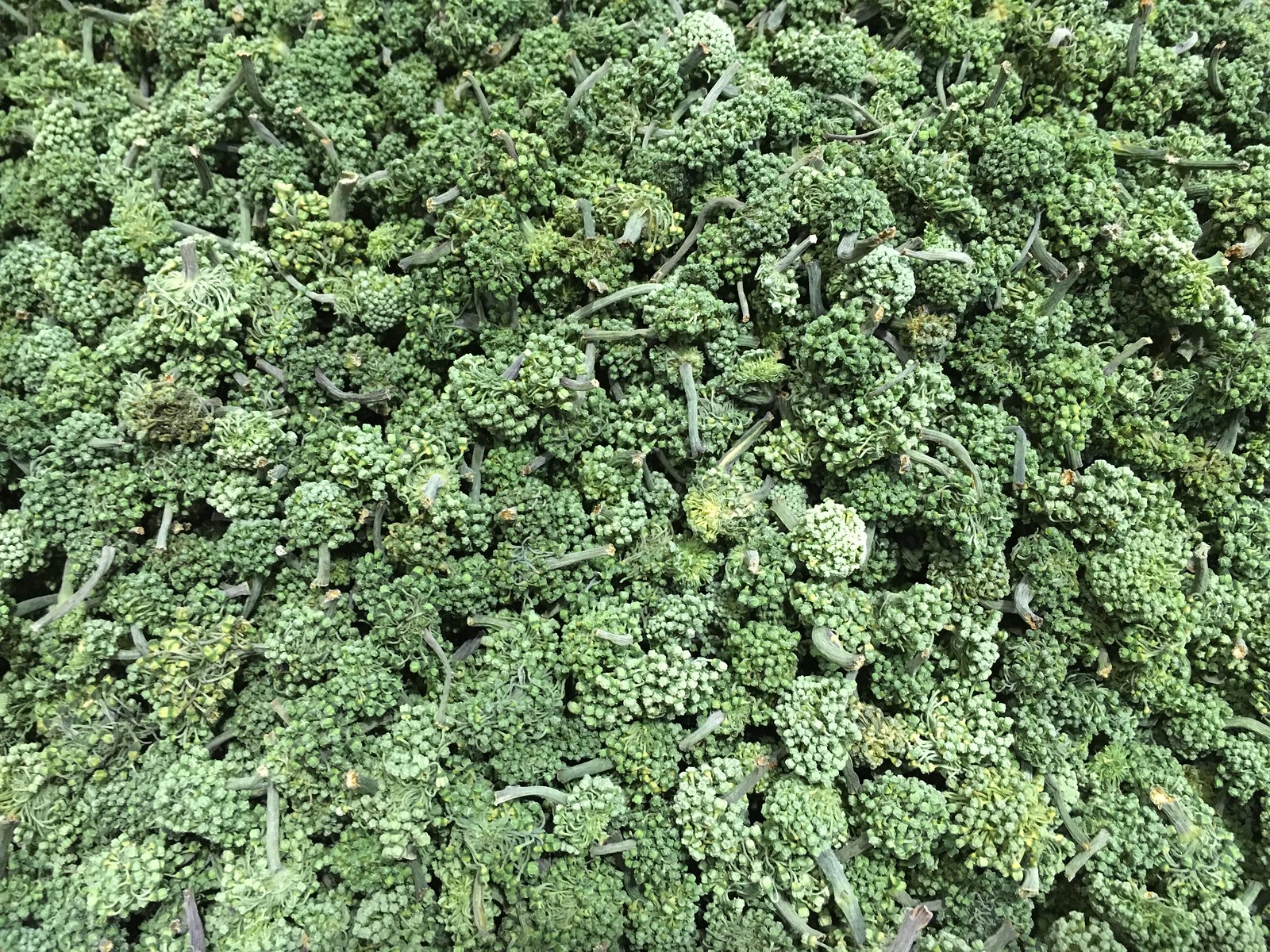This image captures a close-up, tightly packed arrangement of broccolini, filling the entire frame in a lush, verdant display. Known for their long stems and small florets, the broccolini appear in various shades of green, ranging from nearly white to deep, rich green. The intensity of the bright lighting suggests the image was likely taken with a flash or under strong natural sunlight, which highlights the intricate details of the vegetable. Some crowns show a hint of yellowing, suggesting optimal freshness. With their identifiable stems and intact crowns standing out prominently, the broccolini creates an almost forest-like impression, making it challenging to discern scale without a point of reference. The densely packed broccolini stretches across the entire photograph, leaving an impression of a vibrant, green landscape.